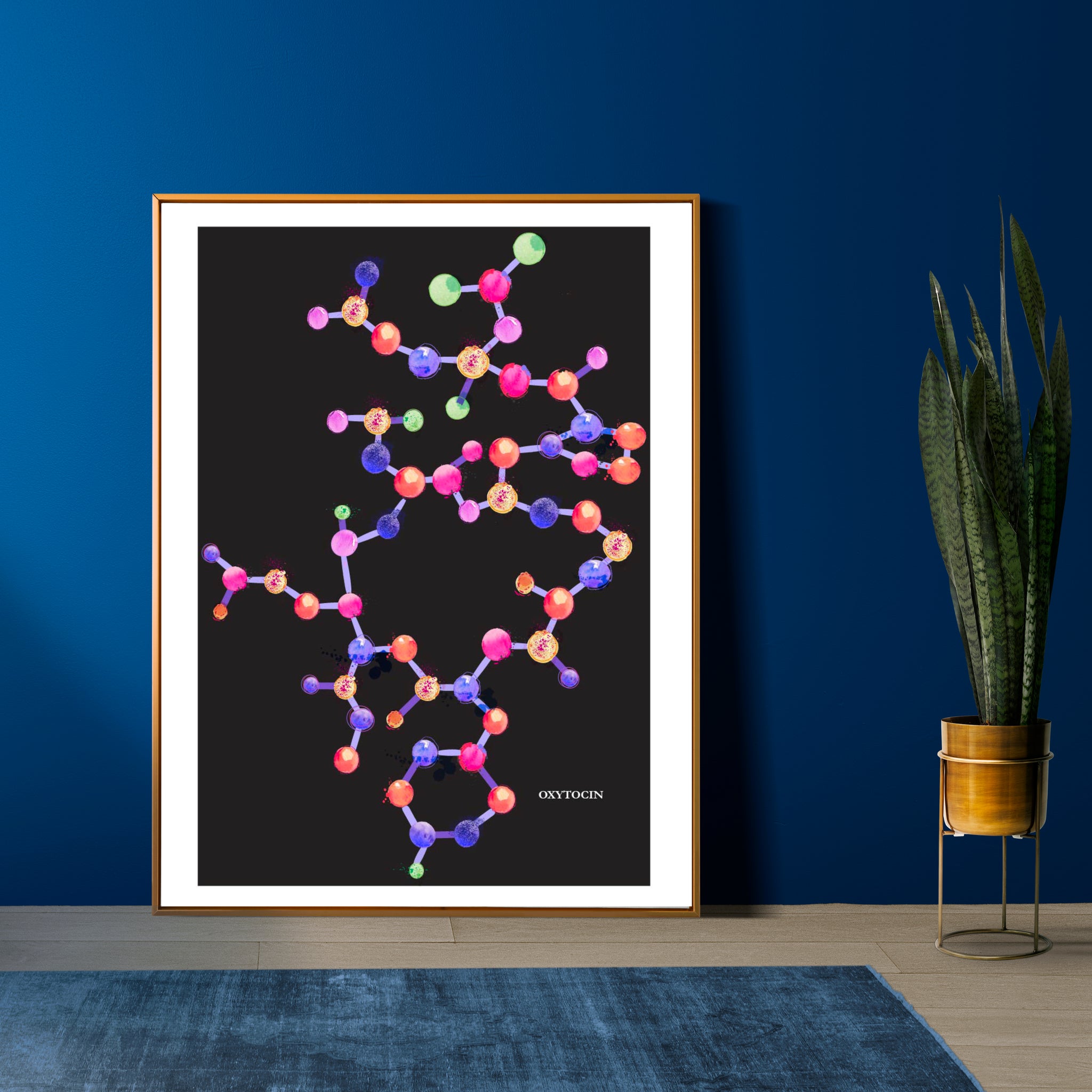The image depicts a framed painting of the chemical structure of oxytocin, leaning against a dark navy blue wall. The painting features a black background with a detailed illustration of interconnected molecules in various colors, including green, purple, pink, blue, and yellow, connected by small rods. The word "oxytocin" is written in smaller white text in the bottom right corner of the painting. It is framed with a gold trim and white matting. To the right of the painting is a tall green plant with long fronds, housed in a small brown pot with a yellow bottom, set inside a brass-colored holder. The plant stand adds height and contrast to the composition. The floor is a light wood vinyl laminate with a lighter blue rug partially visible in front of the painting, adding texture and color to the overall scene.